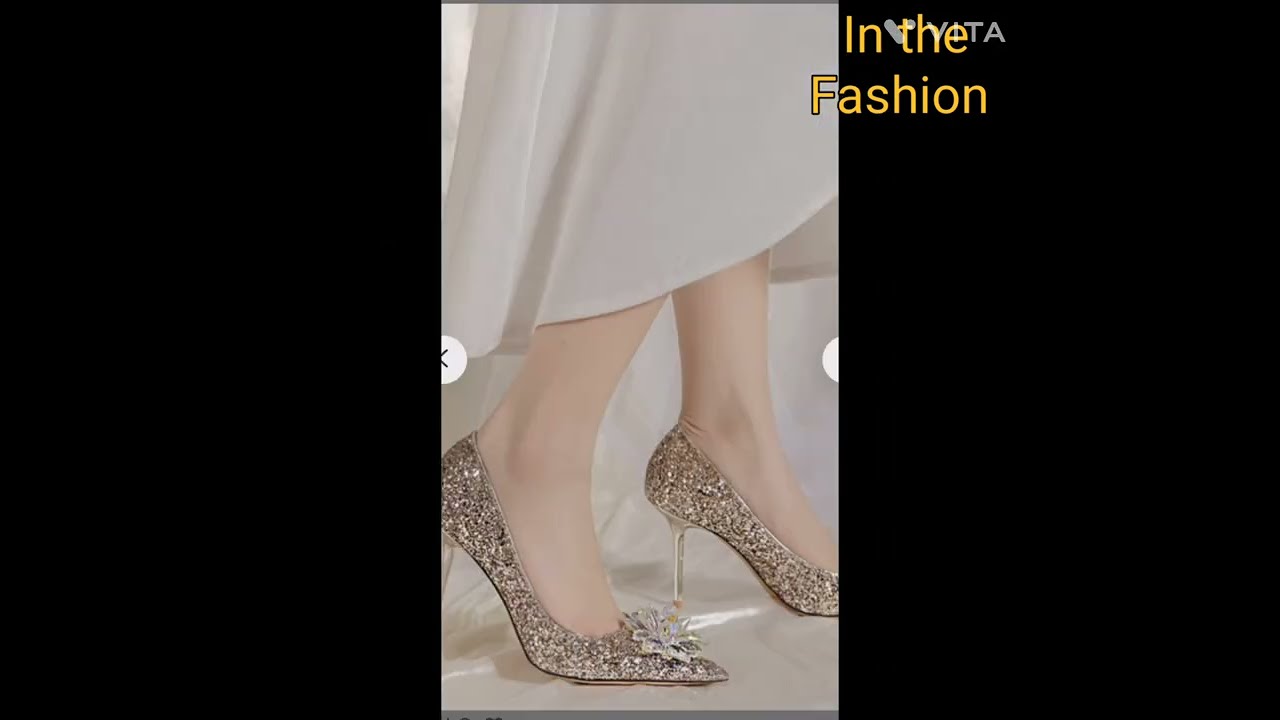The image features a close-up of a woman's lower legs and feet, showcasing her vibrant, glittering high-heeled shoes adorned with sparkly rhinestones or gemstones and a decorative flower on the toe. The shoes are a mix of goldish-silver or champagne color and are the focal point, suggesting an advertisement for the footwear. The woman is bare-legged, wearing a long, flowing white or off-white dress that reaches down to her shins. She stands facing right, against an off-white background, on a similarly colored surface. The photograph is centered within a horizontal rectangle flanked by black vertical borders on each side. At the top of the image, yellow text reads "In the fashion," with some barely visible gray text behind it. The overall scene is light and muted in color, emphasizing the sparkle and detail of the heels. Arrows on each side hint at the option to scroll through more images.